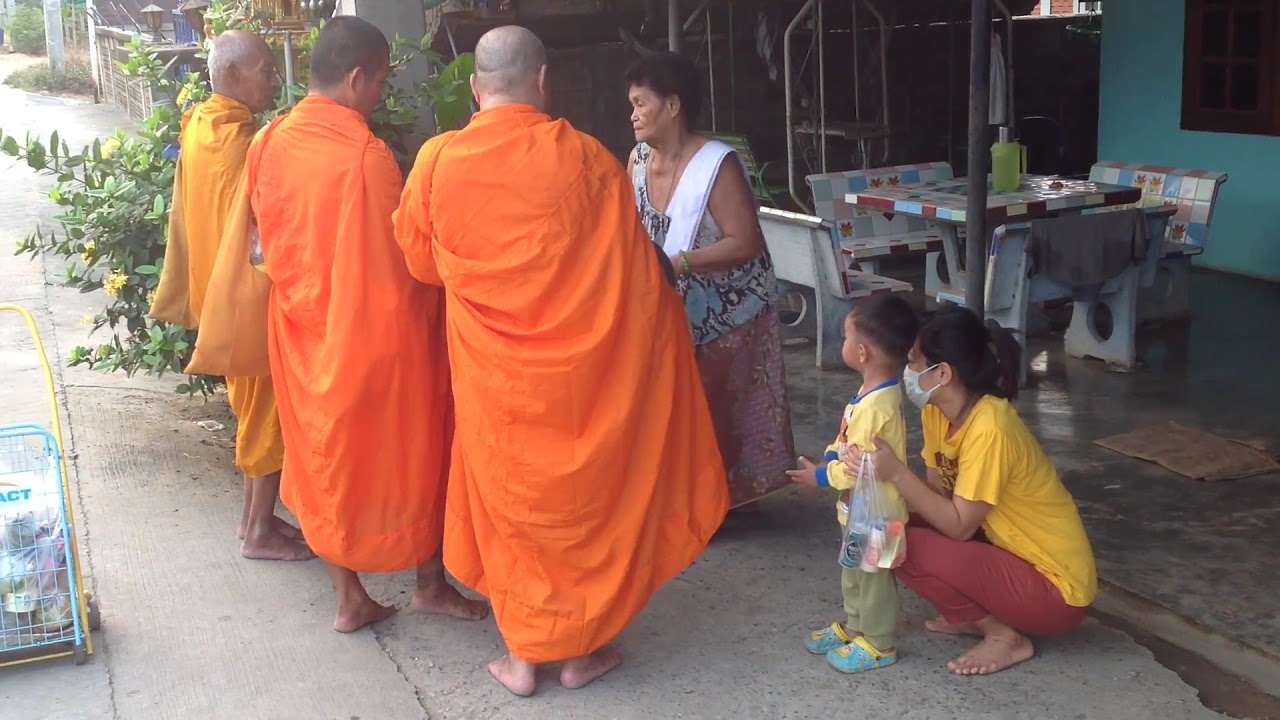In this outdoor photo, three Buddhist monks, dressed in bright to light orange robes, are engaging in a conversation with an elderly Asian woman seated on a stone pavement. The monks, with shaved heads and bare feet, contrast slightly in their appearance with one bald, one almost bald, and the third having some hair. The older monk is shown in profile, while the younger two are seen from the back. To the right of the monks stands a little boy, around two or three years old, wearing a yellow shirt, green pants, and blue crocs. Crouching nearby is a young woman, likely the boy's mother, dressed in a yellow t-shirt, red pants, and holding a plastic bag. She wears a face mask and is also barefoot. In the background, there is a table with four chairs and a green bush, suggesting a porch setting. Additionally, a shopping cart with the letters "ACT" can be seen behind the monks. The scene captures an interaction in an Asian country, marked by varied colors such as gray, yellow, light blue, maroon, and shades of green, all under the midday light.